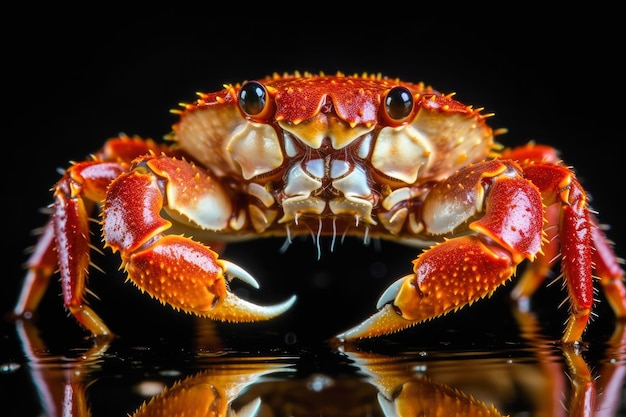This stunning close-up photograph captures a vivid, reddish-orange crab standing on a reflective surface, revealing a mirrored image below it. The crab is positioned facing directly towards the camera, making its two black, beady eyes prominently visible. The high-resolution image showcases the detailed texture of the crab's exoskeleton, highlighting the numerous small spikes and fine white hairs that cover its body. Its claws, legs, and various joints are intricately defined, with a noticeable gradient of colors—yellow hints on its claws and legs, and subtle white and pink shades on its underside. The crab's face, including its mouth parts, is well-illuminated and clear, featuring light reflections that enhance its realistic appearance. Set against a stark black background, the overall composition ensures that the crab remains the central focus of this highly detailed and lifelike image.